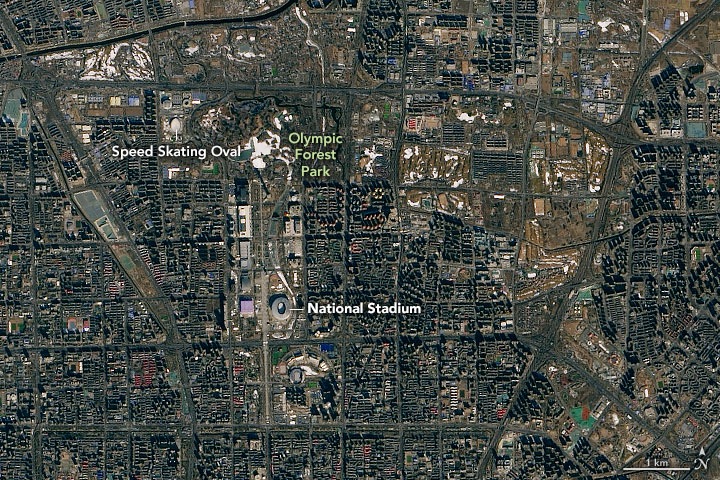This image is an overhead aerial view, likely captured from a satellite or drone, depicting a bustling cityscape with various landmarks labeled. The photograph shows densely packed buildings, intersecting highways, and a grid of streets. Key points of interest include a prominent circular structure marked as the National Stadium in the middle of the image. To the upper left, there is an oval shape labeled as the Speed Skating Oval, and nearby, in light green text, is the Olympic Forest Park. The bottom right corner features a scale bar indicating a distance of one kilometer and a north-pointing compass arrow. The scene is vibrant, with various roads and structures differing in colors, including black, red, blue, and green, suggesting a complex and diverse urban area.